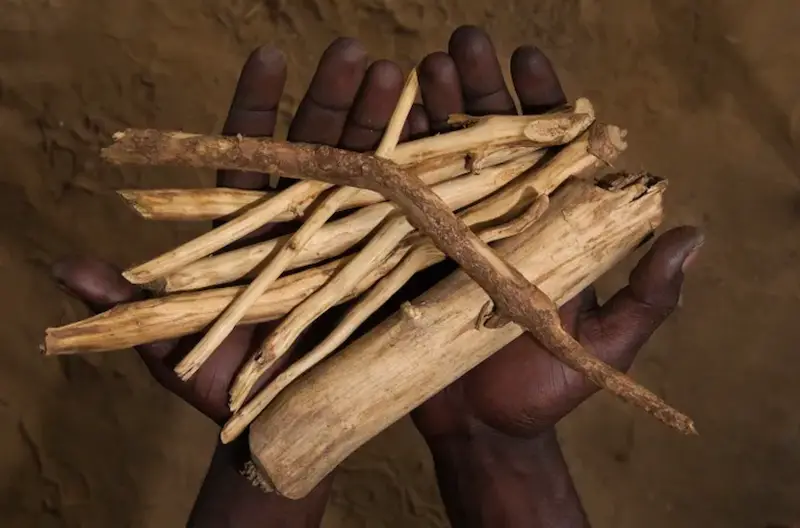In this photograph, we see a pair of black hands holding an assortment of twigs and sticks. The hands are positioned with palms up, meeting at the little fingers, and the perspective is from above, focusing on the hands and their contents. The background, a blurred sandy or sand-like dirt, emphasizes the collection of wood being held. The twigs vary in thickness and length, primarily light brown in color, with a notable darker brown twig that arches slightly across the top of the hands. These gnarled and bent twigs appear to be suitable for kindling, suggesting they are being gathered for a fire. The image captures the intricate textures of both the skin and the twigs, telling a story of resourcefulness against a minimalistic backdrop.